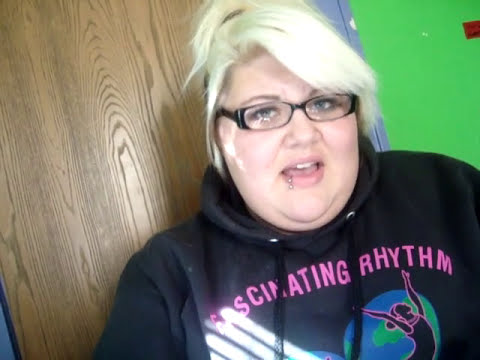The image features a woman with dyed light blonde hair styled into a ponytail bun, with a strip forming bangs covering the left side of her forehead. She has a lip piercing on the lower left corner of her mouth and wears 50s style black-rimmed rectangular glasses. Clad in a black hoodie adorned with pink text that reads "Fascinating Rhythm," the hoodie also features a graphic of a dancer atop a globe. She appears to be speaking directly at the camera, though it's unclear whether she's holding it herself or if someone else is. She is positioned in front of a laminate wood wall that transitions into a bright green wall, with sunlight partially illuminating her. The camera angle is approximately 20 degrees to the left, conveying a slightly tilted perspective.